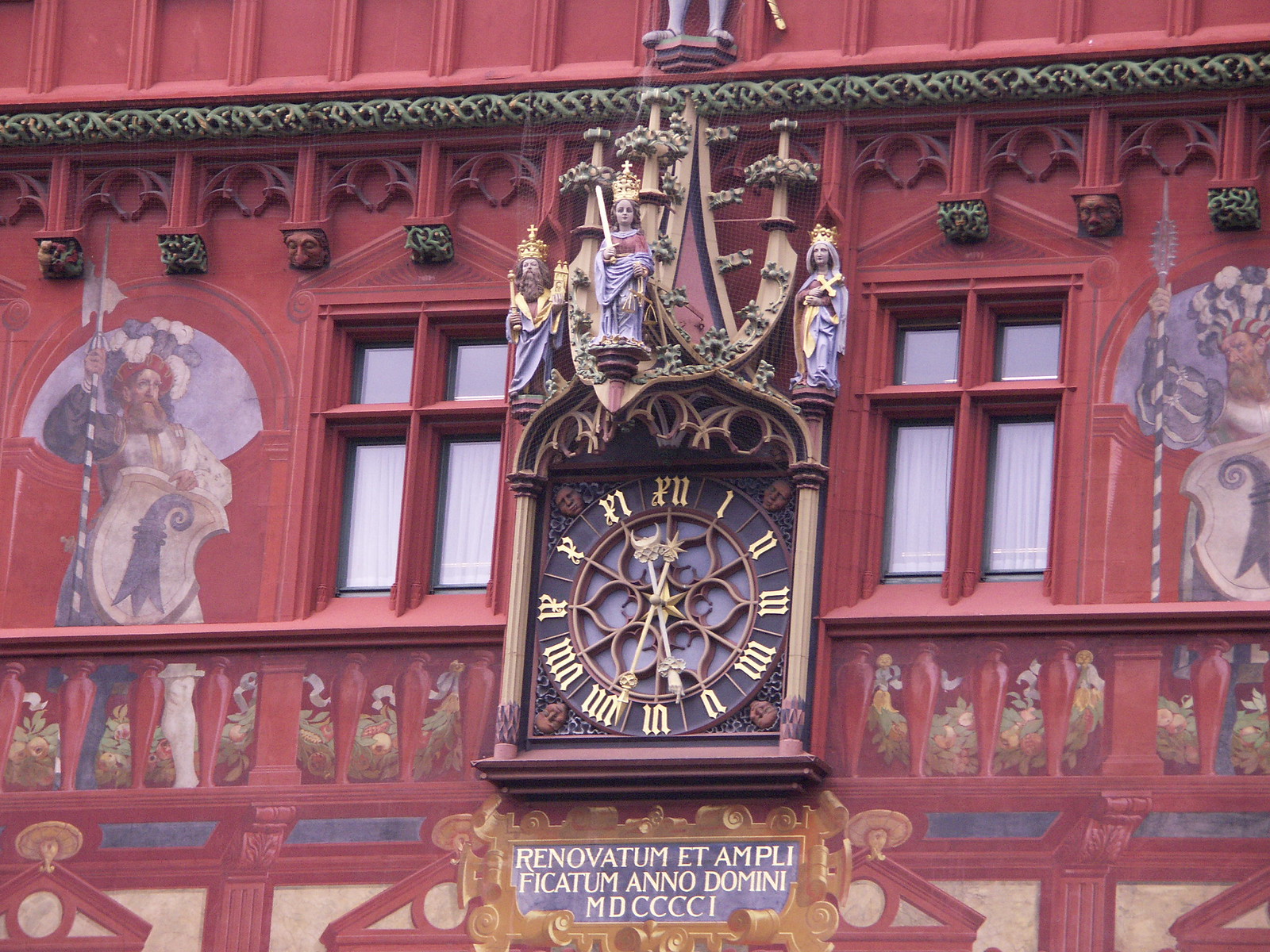This color photograph, taken outdoors in the daytime, fills the entire frame with an ornate exterior of a historical red building that appears to be a church. Dominating the center of the image is a large, square clock with a floral-like center, gold hands, and Roman numerals set against a black circular background. The clock is flanked by two pillars and rests on a gold, shell-like plinth featuring Latin text: "Renovatum et Ampli Fictam Anno Domini M.D. CCCCI," indicating a renovation date in Roman numerals.

Above the clock, an intricate scene unfolds with three-dimensional sculpted figures, including what seem to be angels or religious icons wearing elaborate clothing, and one resembling Mary Magdalene holding a Bible. These figures are positioned atop a small, ornate tower-like structure. On either side of the clock are two windows, accompanied by detailed paintings depicting men in historical tunics, one holding a spear with an axe head and the other a plain spear. These paintings extend across an artificially-painted balcony railing and feature additional elements like flowers and legs of another figure.

The building's exterior is richly adorned with colors including red, green, blue, purple, white, and yellow, enhancing its detailed paintings and architectural features, which emulate elements like bushes, flowers, and a Roman coliseum.